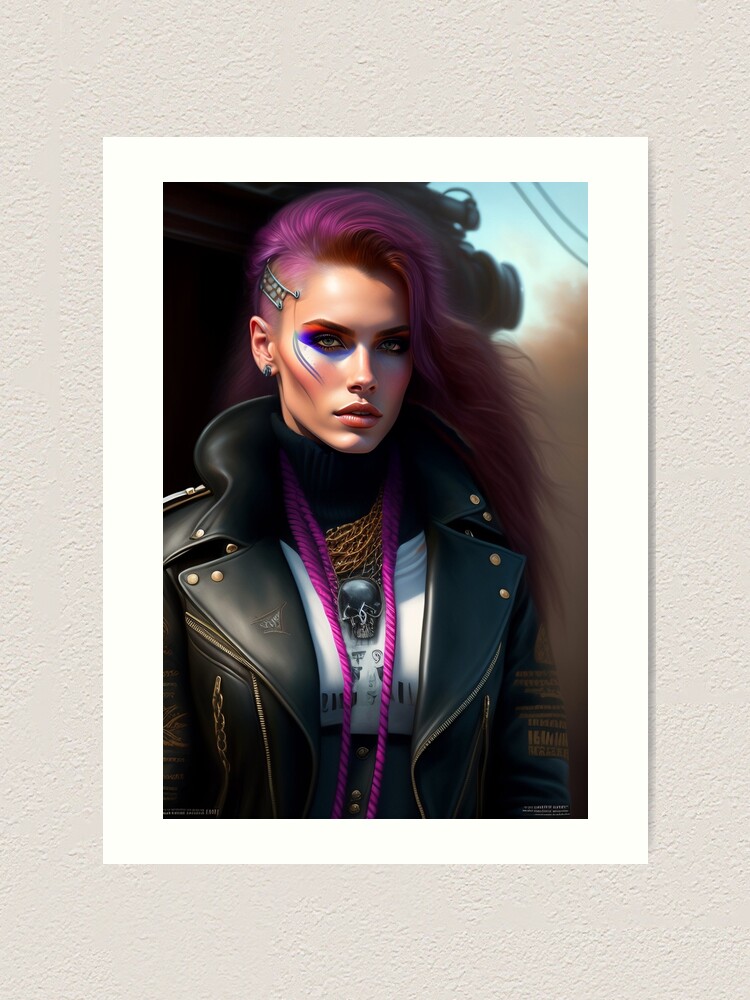The digital painting showcases a highly detailed, semi-realistic image of a woman from the waist up, set against a blurred background with hints of blue sky and tree-like structures. Framed within a white rectangular border, the composition is against a gray patterned background. The woman has striking long purple hair with one side of her head shaved, adorned with a metal brooch. She also has locks of pink hair cascading to the front. Her makeup is bold, featuring heavy blue eyeshadow on the lower lids, orange eyeshadow on the upper lids, and accentuated with blue stripes painted near her eyes. Her light skin contrasts with the vivid makeup.

She is dressed in an elaborate black leather jacket, embellished with gold brads, buttons on the collar, and zippers. Underneath the open jacket, she wears a white t-shirt, alongside a thick black belt. Multiple necklaces adorn her neck, including gold chains and a distinctive violet cord, as well as a skull pendant. She also seems to sport a black turtleneck beneath all this, adding layers to her edgy yet intricate ensemble.